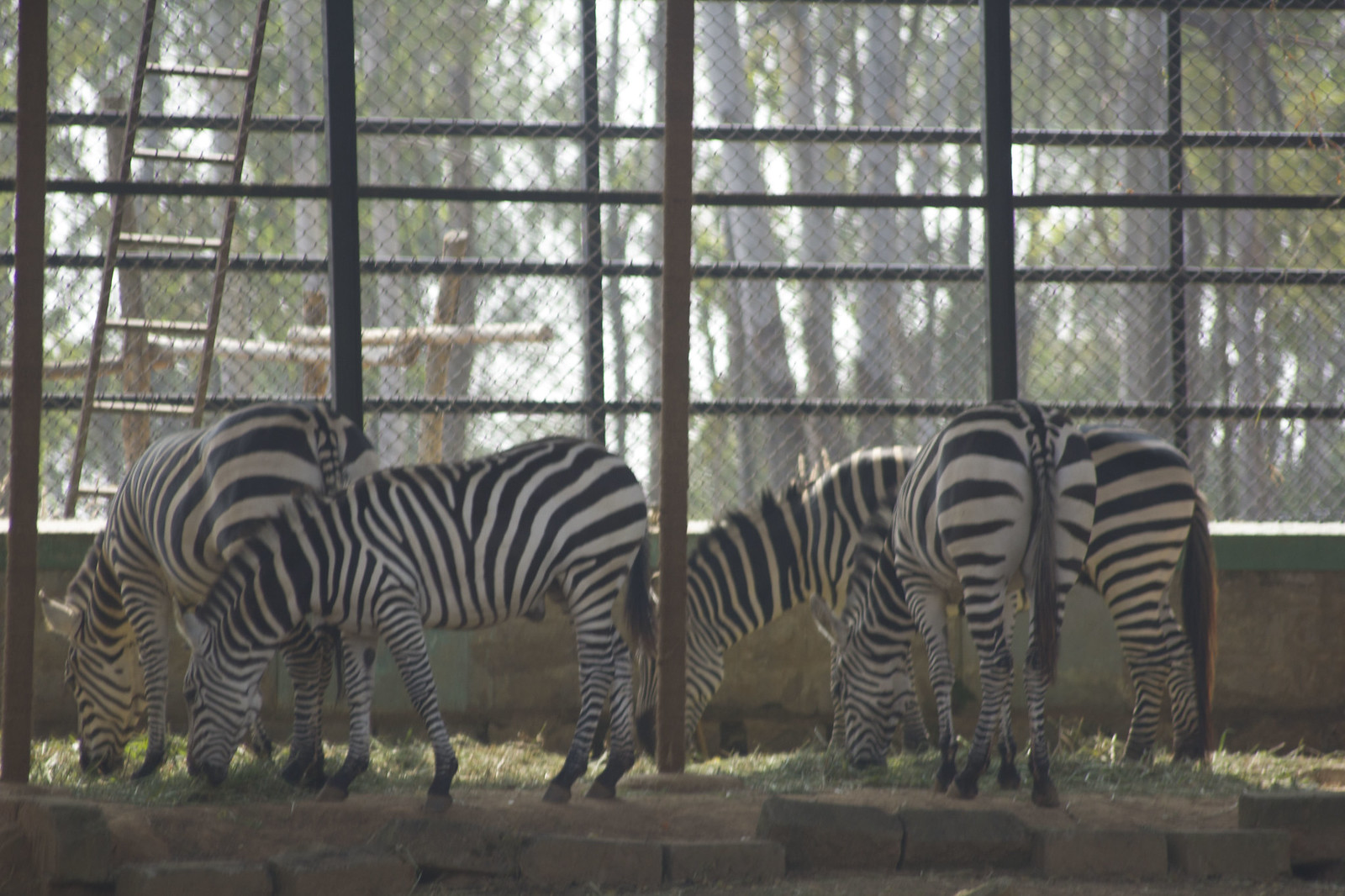This is a horizontal, realistic color photograph taken at a zoo, depicting four adult zebras inside a shaded enclosure. The zebras, adorned with their traditional black and white stripes and long black tails, are all oriented towards the left of the image, with their heads bent down, seemingly grazing on the straw intentionally left for them. The enclosure features supportive pillars and a brick floor, alongside a chain link fence with bars that separate it from the outdoors. Beyond the fence, a picturesque scene with tall, brown trees and green leaves against a white sky is visible, contributing to a forest-like backdrop. A wooden ladder is propped up against the left side of the structure, enhancing the rustic atmosphere of the animal barn. The absence of people or motorized vehicles emphasizes the zebras' undisturbed state.